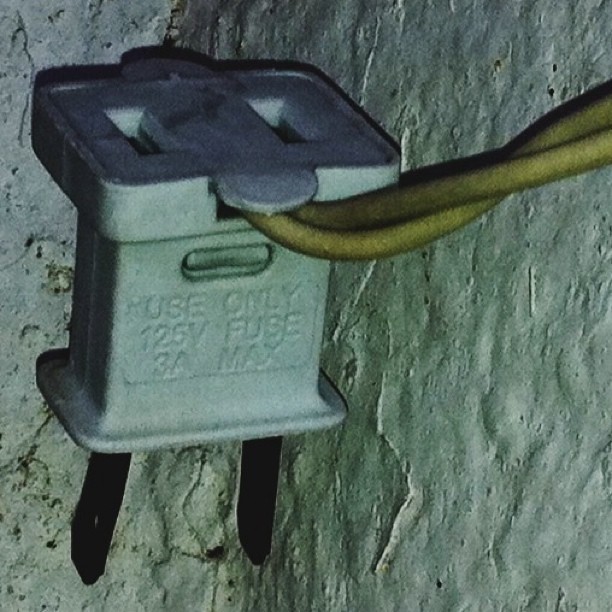The image depicts a close-up of a white plug adapter. The adapter has indented text on its side that reads, "Use Only 125 Volt Fuse, 3A Max." This adapter converts a three-prong plug to a two-prong plug, with the two prongs visible at the bottom. Emanating from the adapter are two thick, intertwined yellow wires that twist upwards and out of the frame. Behind the adapter is a rough, off-white or grayish concrete wall, which appears weathered and old, suggesting the setting is likely an unfinished basement or garage. The wall features cracks, patchwork, and small holes, adding to its aged appearance. The overall scene gives a utilitarian and slightly deteriorated look.